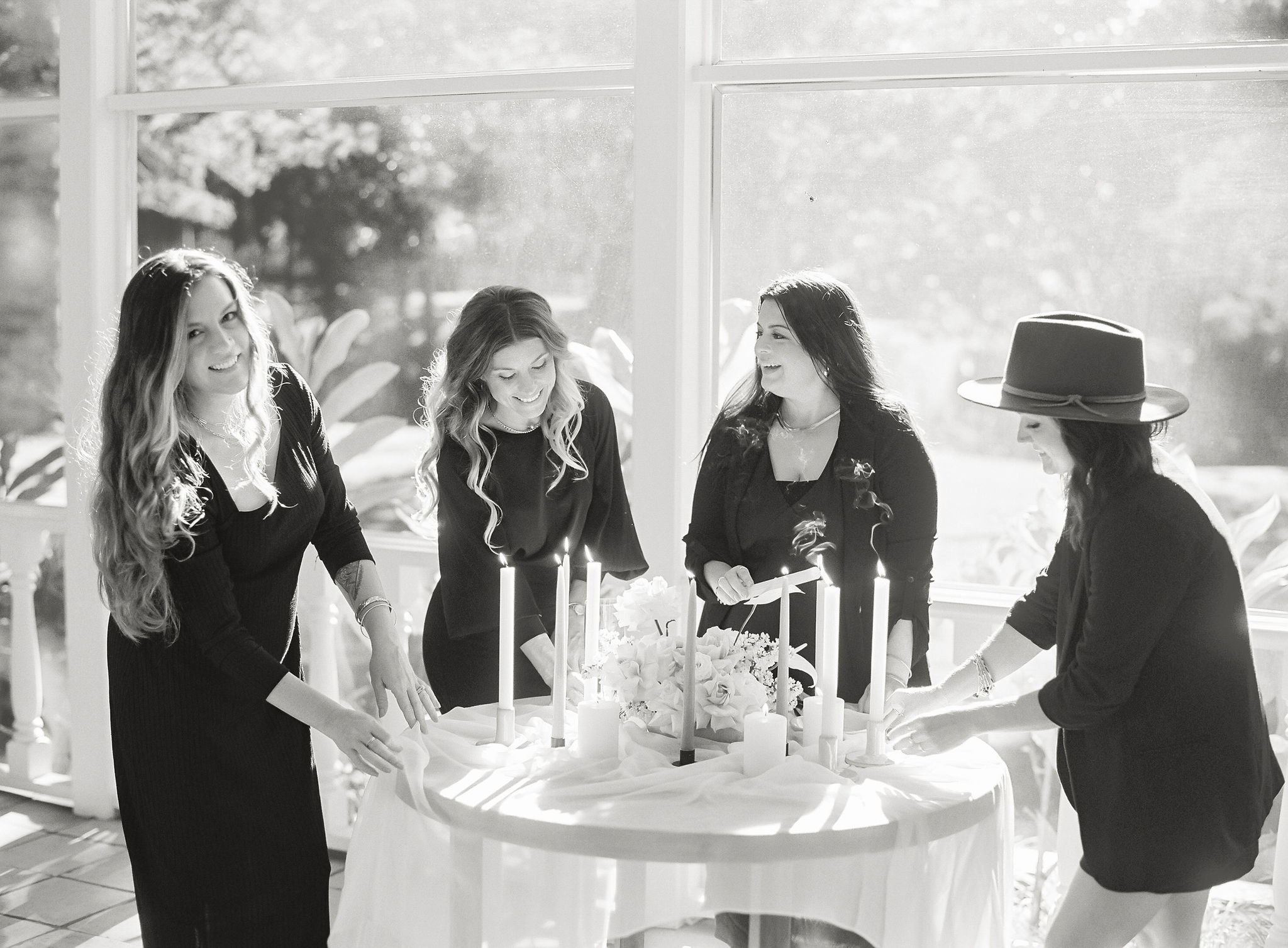In this detailed black and white photograph, four women, all dressed in black outfits, are gathered around a circular table covered with a transparent tablecloth. They appear to be diligently preparing the table, setting and lighting candles, which are already lit. At the center of the table rests a beautiful white floral arrangement. Each of the women is engaged in different tasks around the table, with one woman on the left smiling towards the camera. The image is clear and bright, benefitting from the natural light streaming through large floor-to-ceiling picture windows that reveal a view of trees outside. The setting suggests a venue prepared for a special occasion, possibly a wedding, with its elegant decor and meticulous arrangement. The backdrop includes white railings and ample foliage visible through the expansive windows, adding to the serene and picturesque ambiance of the scene.